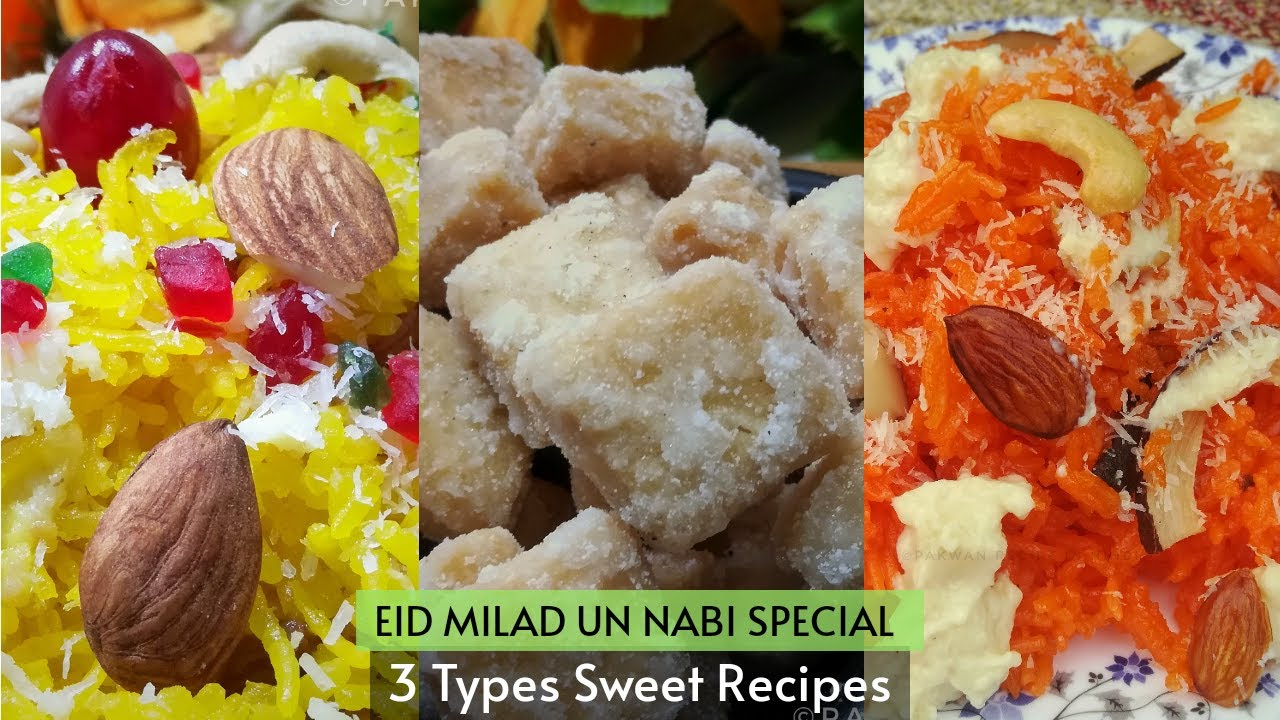This landscape-format photograph showcases three different sections, each featuring a type of sweet traditionally made for Eid Milad un Nabi, the celebration marking the end of a Muslim fasting period. The accompanying text reads "Eid Milad un Nabi Special, three type sweet recipes," highlighting the cultural significance of these dishes.

The left section presents a vibrant dish of yellow rice, garnished with candied fruit, almonds, and cherries. The central section features what appears to be bite-sized square sugar cookies or possibly pieces of dough encrusted with sugar or cinnamon, offering a tantalizing glimpse of their crumbly texture. The right-hand section displays a rich and vibrant carrot halva adorned with grated orange, almonds, cashews, and a sprinkling of coconut, enhancing the visual and flavor complexity. Together, these images form a mouthwatering tableau of sweet delicacies emblematic of Eid celebrations.